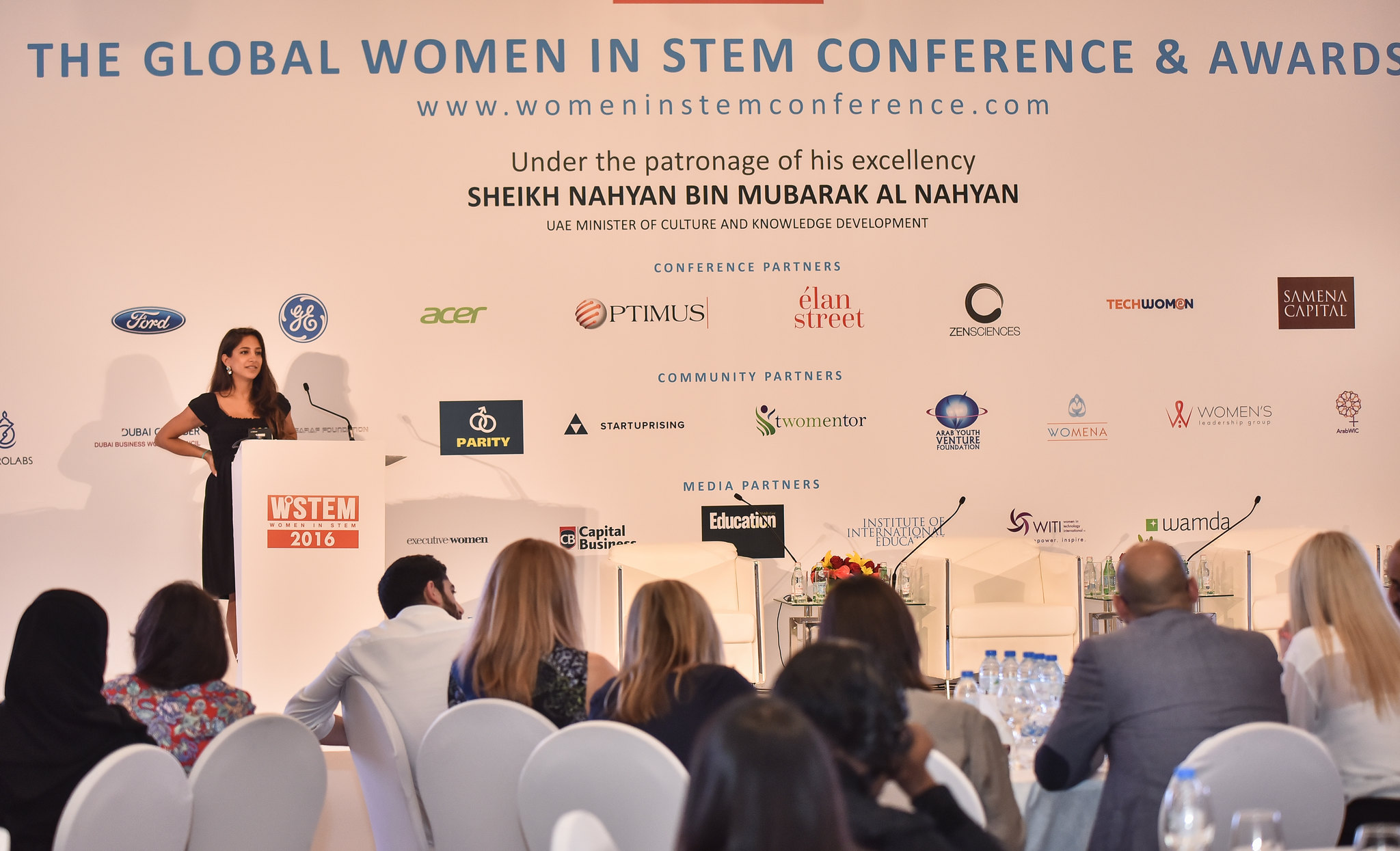The image captures a scene from the Global Women in STEM Conference and Awards 2016. At the forefront, a woman in a black dress stands confidently at a white podium, which features the text "WSTEM" in white and an orange rectangular area stating "2016." She is addressing the audience with a microphone, her right hand placed on her hip. Behind her, the stage is bordered by a light gray wall adorned with numerous sponsor logos, including Ford, GE, Acer, Elan Street, Optimus, Tech Woman, Semina Capital, Community Partners, 2Mentor, Startup Rising, Parity, Education, Media Partners, Capital Business, and Wynn. Above these logos, in large blue text, the banner reads “The Global Women in STEM Conference and Awards,” followed by the website www.womeninstemconference.com. The attendees, mostly women with a few men, are seated in white chairs, their heads turned towards the speaker. The ambiance is professional and focused, with the audience intently engaged in the presentation.